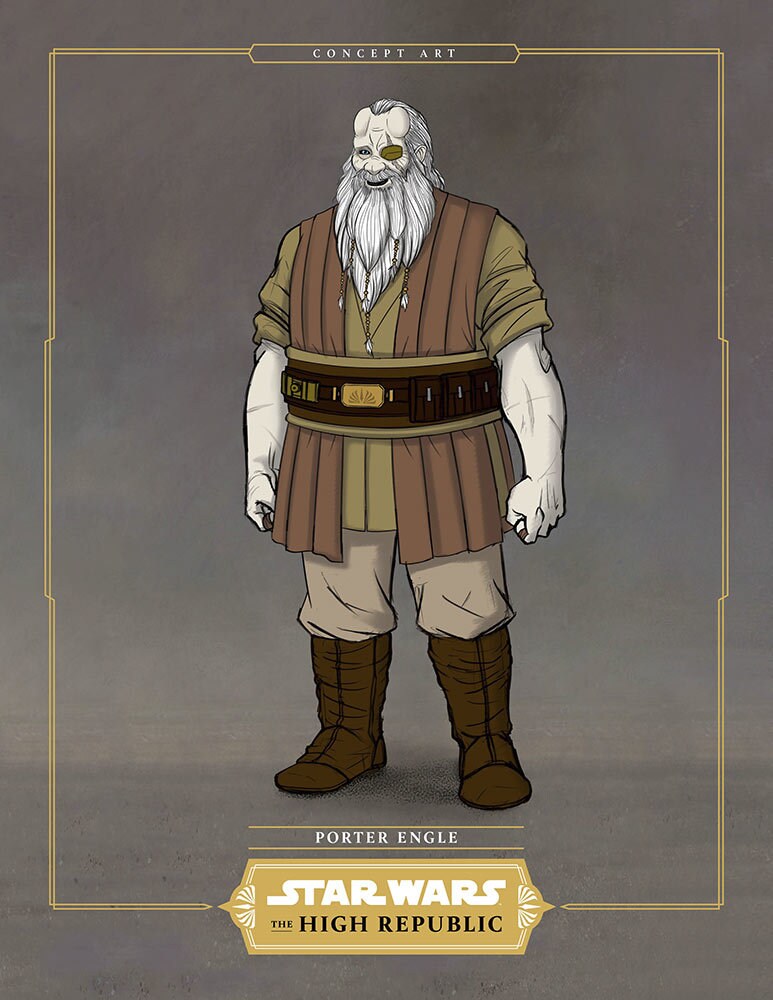The image is a detailed concept art of a character from "Star Wars: The High Republic," set against a gray, smoky, and tan colored background, resembling a poster. A prominent yellow border frames the image, connecting to a banner at the bottom that reads "Star Wars: The High Republic" in white text on a gold and white plate. Just above the banner, in white text flanked by two thin gold lines, the name "Porter Ingle" is displayed.

Porter Ingle, portrayed in a cartoonish, animated style, stands as a stout, strong man. He has a long white beard adorned with beads, a white mustache, and long white hair combed back. A notable scar bisects his left eye, which is covered by a brown eye patch, giving him a rugged appearance. He is dressed in a Star Wars-inspired outfit reminiscent of Anakin Skywalker's attire, including a greenish-tan shirt with rolled-up sleeves, layered with a brown vest, and accessorized with a large belt around his upper waist. He completes the look with khaki pants and brown high-rise boots. The overall presentation is vibrant and detailed, capturing the essence of a heroic, seasoned character from the Star Wars universe.